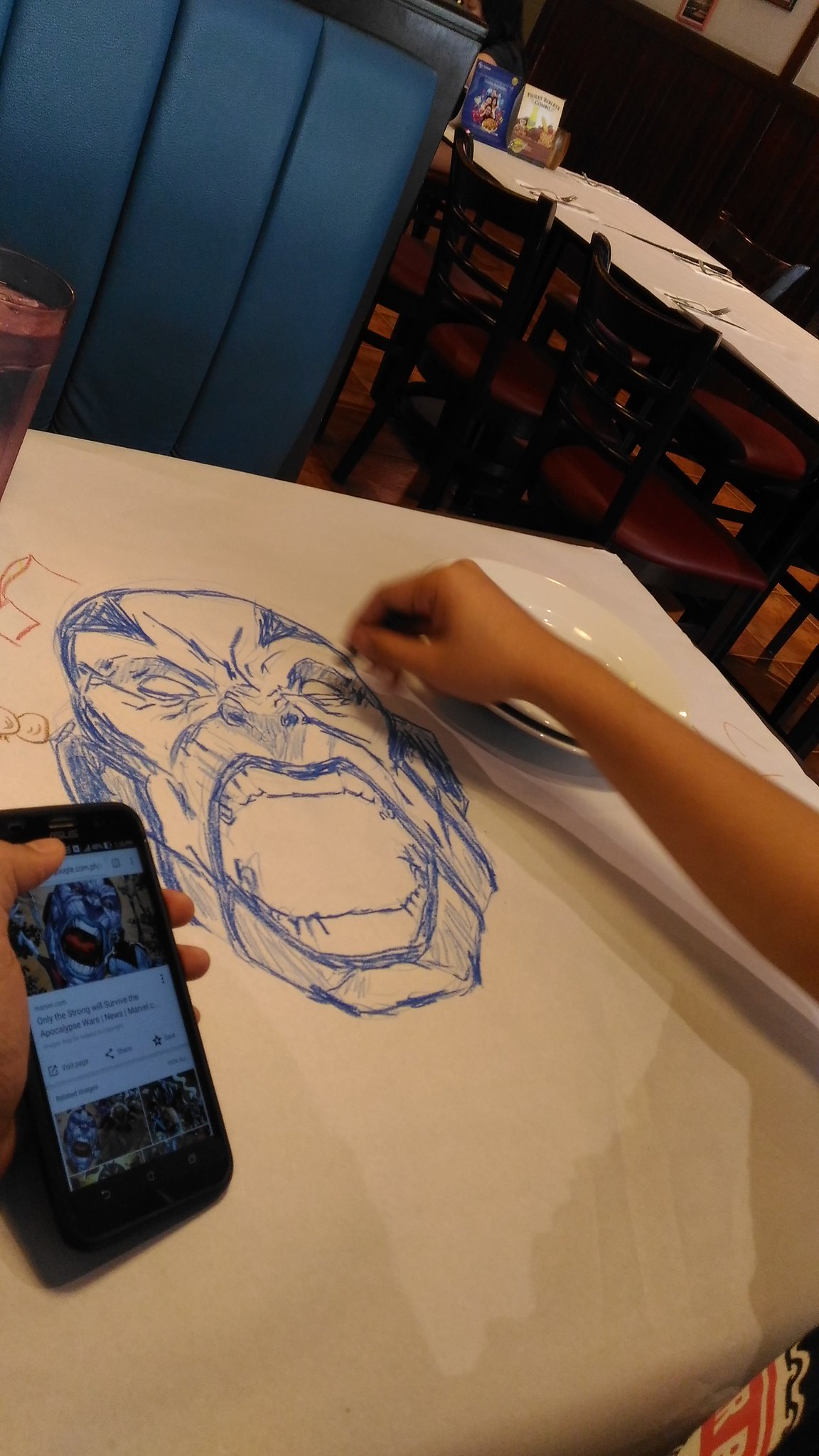In this detailed image captured inside a restaurant, we observe a uniquely covered table adorned with white sheets of paper, a feature that encourages patrons to unleash their creativity using provided crayons. Central to the scene is a young child engrossed in drawing a character from the Marvel universe with a blue crayon. The character depicted has an angry expression with its mouth open wide. The child is multitasking, holding a smartphone in their left hand, which displays a reference image for their drawing. The phone screen prominently features a text that reads, "Only the strong will survive the apocalypse wars news" followed by "Marvels Comics," though the text is partially cut off. Impressively, the child's drawing closely mirrors the reference image, showcasing their attention to detail and artistic skill.